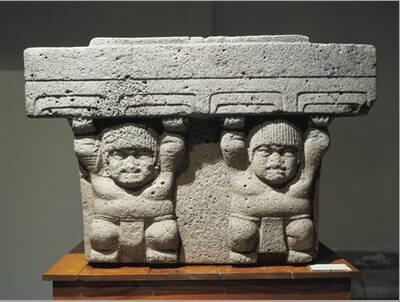The image features a detailed, weathered stone sculpture displayed on a polished, amber-colored wooden table. The sculpture depicts two stout, squarish-shaped figures resembling sumo wrestlers, with intricate carving showing them wearing loincloths and possibly helmets or stylized hair. Both figures are in a crouched position with their arms raised, as if struggling to support a smooth, horizontal slab of stone above them. The men's noses appear to be eroded or broken off. The upper stone slab displays squiggly lines along its lower edge with a groove running horizontally across it. A museum label is attached to the bottom right corner of the wooden table. The background of the photograph is a gray wall.